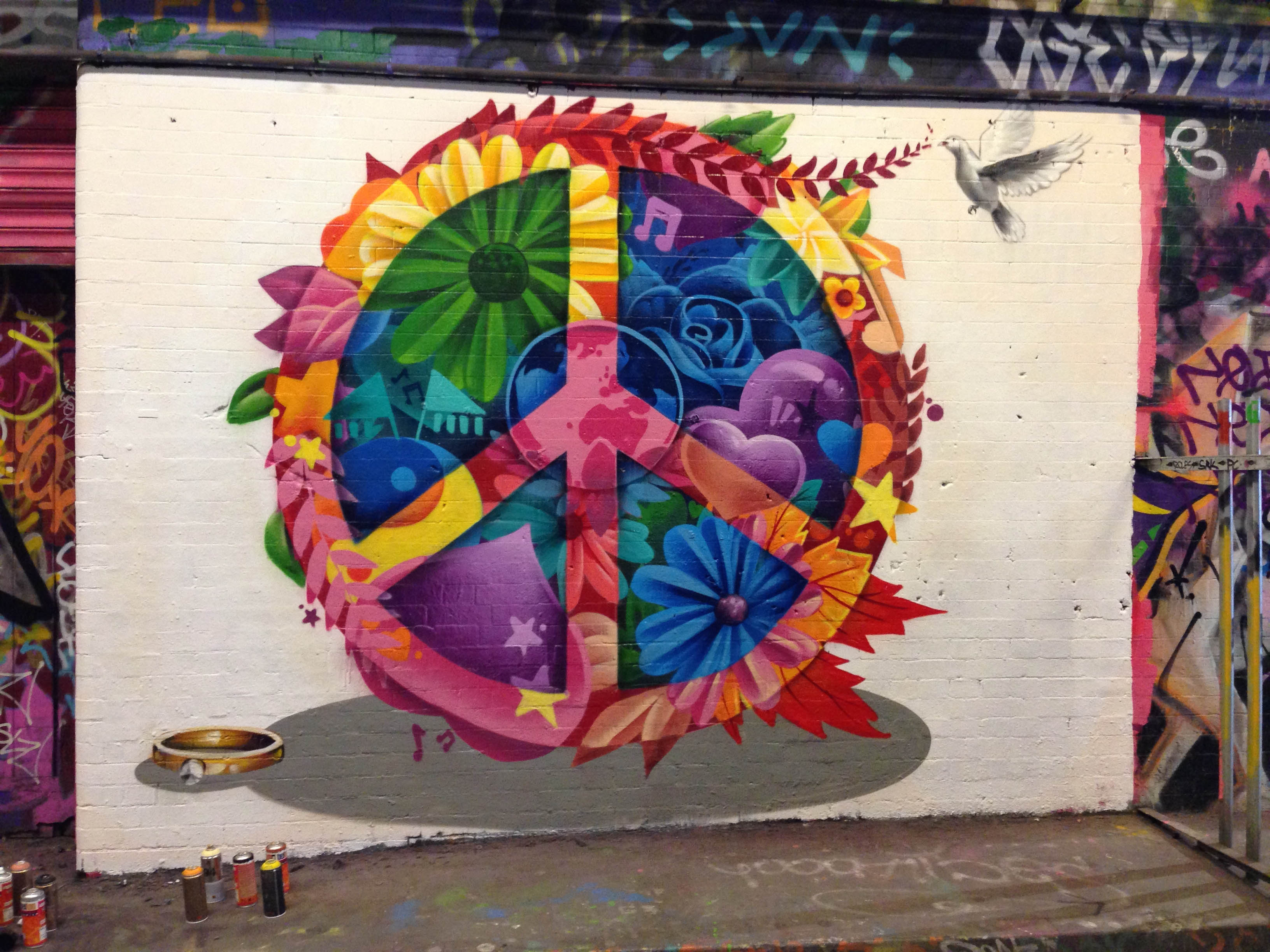The photograph depicts a vibrant, freshly painted mural on the side of a brick building. The central focus is a large, multicolored peace sign with intricate details. Inside the peace symbol, colored in red, yellow, pink, and orange, there are various peace-themed elements: a blue and green Earth, hearts, stars, flowers, and musical notes in shades of blue, green, yellow, and purple. A white dove flies upwards, touching an olive branch that forms part of the circular peace sign with its beak. Surrounding this main image, the brick wall is adorned with an array of graffiti in various colors and styles. In the bottom left of the mural, outside the white rectangular section, there's a ring or tambourine, and in the bottom right, just outside the mural, a collection of paint cans is present.